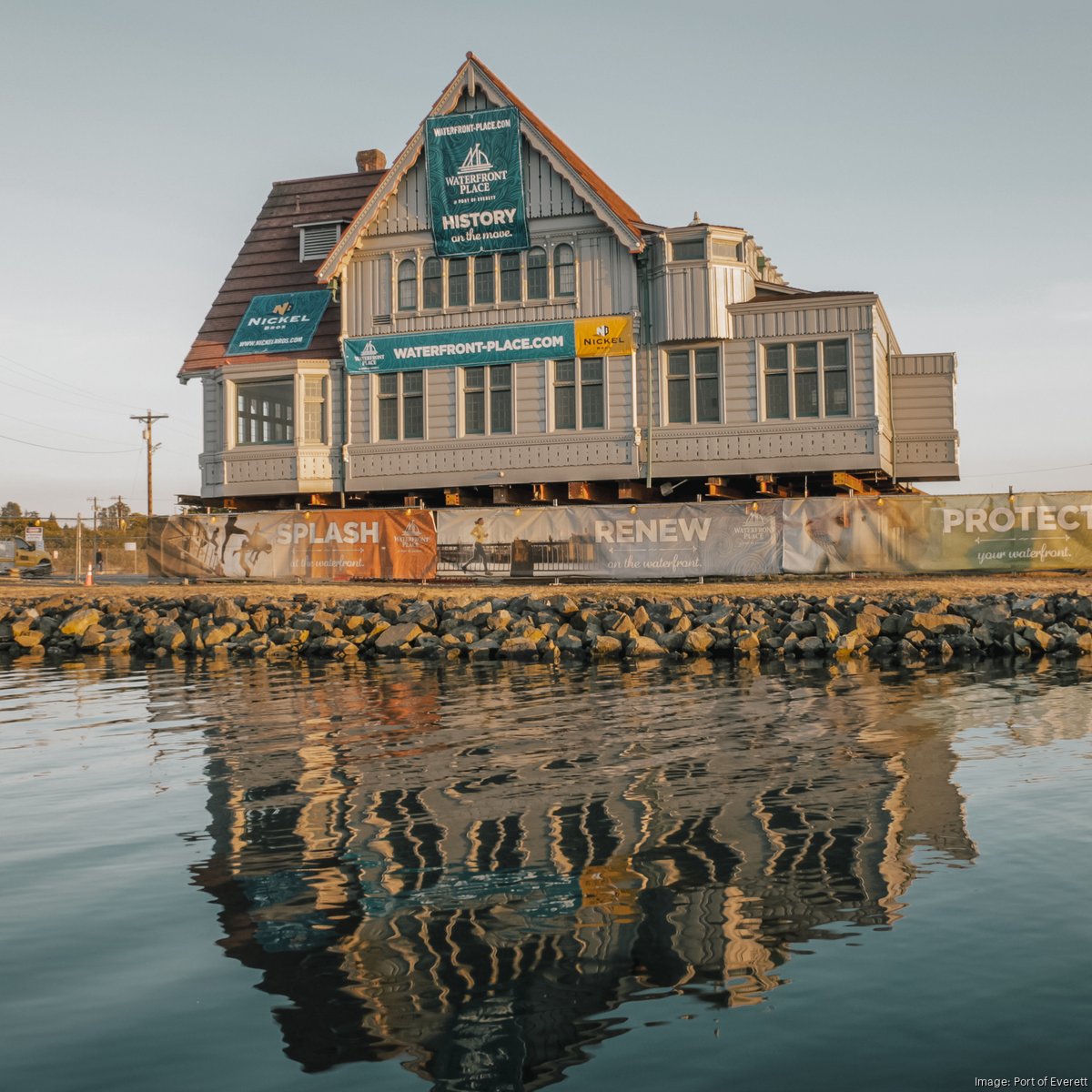This detailed outdoor photograph captures a tranquil lakeside scene. Central to the image is a large, tan-colored Victorian-style building perched on a short, rocky shoreline that resembles a retaining wall. The calm lake beautifully reflects the structure. The two-story building, elevated on stilts with a sloped roof, sports a series of arched windows on the second floor, while larger square windows dominate the first floor. A dormer juts out from the side of the first floor on the right, complementing a lower attached structure on the left that features a bay window and a sloping roof with a small dormer and chimney. Signage is prominently visible around and below the structure, including banners and signs that say "nickelwaterfrontplace.com," "splash," "renew," "protect," and "history," with small icons like a boat and phrases emphasizing play, building, and the environment. Morning sunlight bathes the scene, casting a warm glow from the right, while a telephone pole and other structures stand to the left of the building. The picturesque setting, combined with the serene water and detailed architecture, evokes a sense of peaceful history and community by the lakeshore.